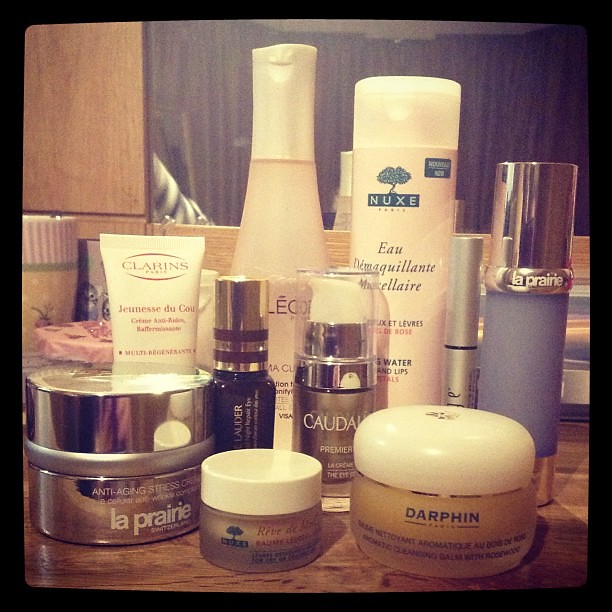The image showcases an array of beauty products meticulously arranged on a brown counter. On the left, there is a jar labeled "Anti-Aging Stress Cream" from La Prairie. Balanced atop this jar is a sleek white tube with black text reading "Clarins Jeunesse des Coups." Moving to the right, a spray bottle with an elegant gold cap is positioned next to a smaller black bottle. At the bottom of the frame, a jar with a white cap reveals a brown paste inside. This jar is flanked by a larger, yet similar jar. The background displays a series of taller white spray bottles, with one prominent blue bottle featuring a silver cap at the far right. The products are set against the backdrop of a wood-paneled wall, complemented by a mirror that adds a touch of sophistication to the scene.